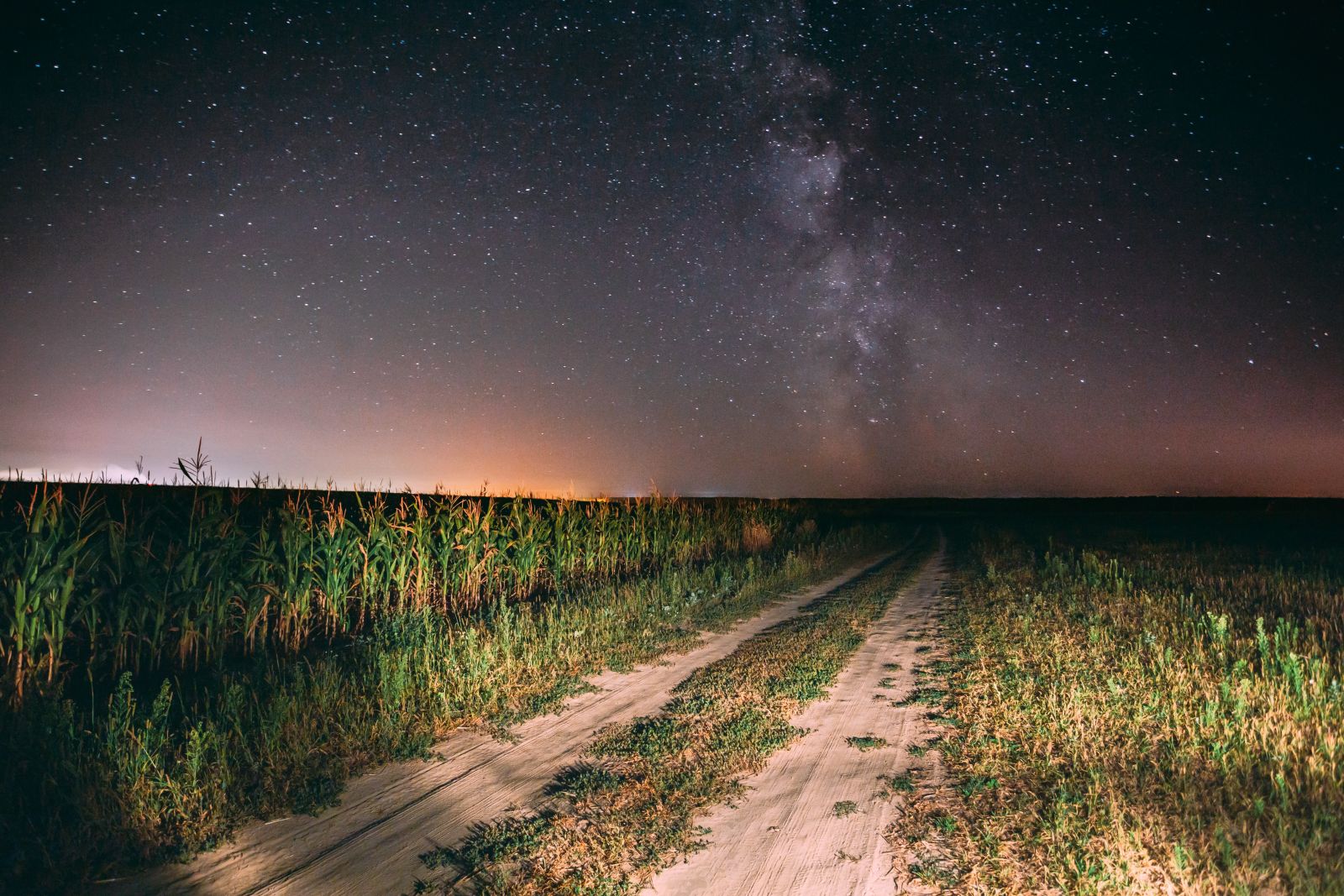Under a star-studded night sky, a serene dirt country road stretches out into the foreground of the image. The road, dotted with patches of brown and green, has a line of withered grass running down its center. On either side, lush green grass grows abundantly, and the left side is bordered by what appears to be a cornfield with young shoots sprouting from the soil. The horizon is bathed in soft shades of peach, white, and a delicate blend of pink and purple, fading into light gray, purple, and black as it ascends into the sky. This transition is punctuated by the shimmering glow of countless stars, with the Milky Way galaxy's arms streaking vividly across the celestial expanse. The scene is illuminated by the headlights of a vehicle emerging from the lower right corner, adding a warm light to the immediate landscape. In the backdrop, city lights or perhaps distant farm structures add subtle illumination to the far reaches of the field, enhancing the sense of depth and tranquility. The intricate details of the night sky, combined with the rustic charm of the road, create a breathtakingly detailed and picturesque scene.